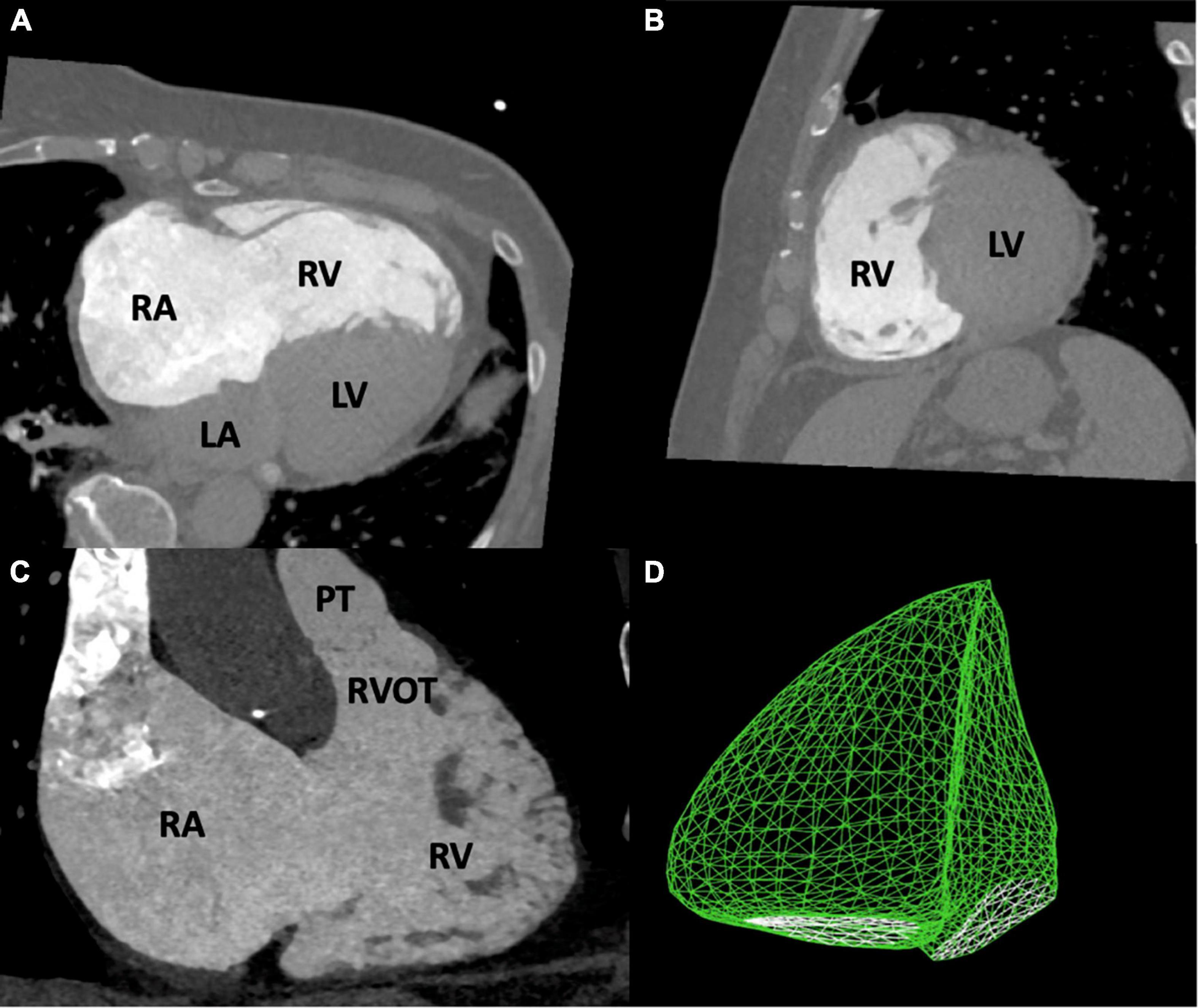This composite medical image presents four distinct panels labeled A, B, C, and D, each showcasing different views and representations of a heart. 

**Panel A** exhibits a black background with a central structure displaying a cross-sectional radiographic image. The structure is divided into quadrants labeled R-A (Right Atrium), R-V (Right Ventricle), L-A (Left Atrium), and L-V (Left Ventricle). The top portion of the mass appears light gray, transitioning to a darker gray at the bottom.

**Panel B** offers a slightly rotated perspective of the same structure found in Panel A. In this view, the light gray region is now on the left while the darker gray is on the right, with the acronyms R-V (Right Ventricle) and L-V (Left Ventricle) labeled accordingly.

**Panel C** provides a side view of the heart, where only specific sections are labeled. The left side of the image marks the RA (Right Atrium), while the right side highlights PT (Pulmonary Trunk), RVOT (Right Ventricular Outflow Tract), and RV (Right Ventricle). This image bears a notable resemblance to the liver in terms of shape and mass.

**Panel D** diverges from the grayscale theme with a vibrant green wireframe model of an oblong, fat, rounded shape that mirrors the heart's structure. This depiction is a graphical representation, potentially generated through a form of medical imaging software, set against a black background without any descriptive labels.

Together, these four panels provide a comprehensive, multi-angled view of the heart, incorporating radiographic imaging and a 3D wireframe model to illustrate its intricate anatomy.